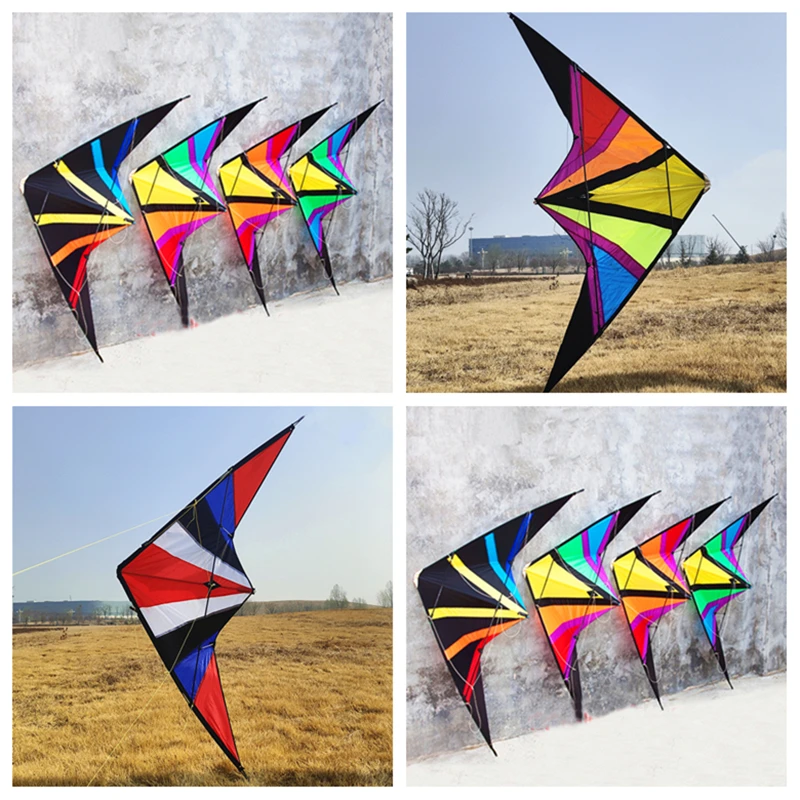This image is a photo collage consisting of four square-format panels arranged in two rows and two columns, separated by white borders horizontally and vertically. Each photo captures different views and arrangements of intricately designed black kites adorned with vibrant stripes and triangles in colors such as red, orange, yellow, green, blue, purple, and black.

In the top left panel, four black kites lean vertically against a gray wall with a whitish-gray ground, their noses pointing towards the wall, displaying wings that stretch outward. These kites form a neat, vertical lineup. The top right panel shows a single kite positioned outdoors in a grassy field with a building in the background. The nose of this kite points to the right, its colorful wings spread leftwards, highlighting its boomerang, bird-wing shape.

The bottom left panel presents another view of a single kite—this time in a similar grassy field but with the nose pointing to the left. This kite also features multicolored stripes and triangles. The bottom right panel mirrors the top left, displaying a slightly different angle of the four kites against the same wall, blending into the photographic representation realism style of the collage.